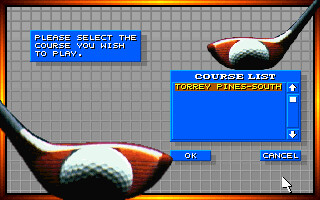The image is a horizontally rectangular screenshot from a golfing video game, featuring a thin border that alternates between yellow, orange, and black. The main background is a gray grid. In the upper right corner of the frame, the lower portion of a golf club is visible with a golf ball positioned in front of it; the club extends diagonally from the upper right down to the left. In the bottom left, a larger, opposite-facing image of a golf club extends from the left side towards the right. In the upper left corner, a small blue rectangular box contains white text that reads, "Please select the course you wish to play." Below the smaller golf club on the right, there is a larger blue box with the text, "Course List, Torrey Pines South." Positioned underneath this box are two buttons side by side, labeled "OK" and "Cancel."